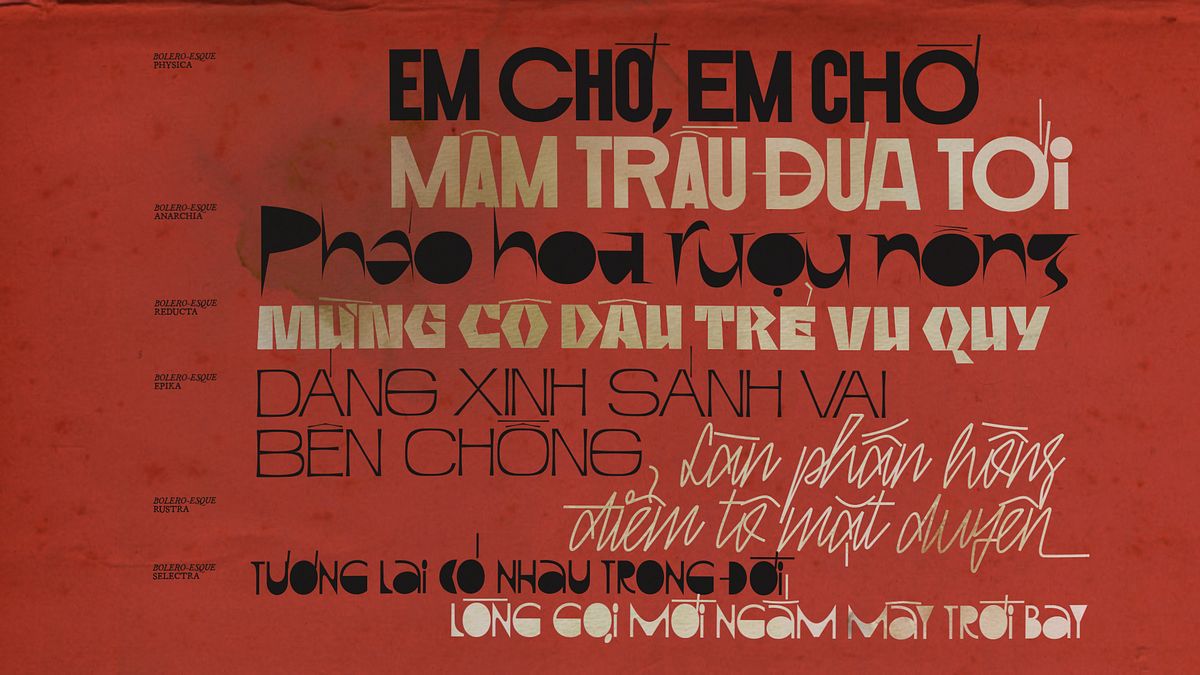The image is a horizontally oriented, color illustration with a background of deep brick red. It features an intricate arrangement of typography in a foreign language, consisting of approximately eight lines of text. The lettering alternates between black and an off-white or cream color. The top line is black, followed by cream, and so on, with each line presenting a different font style and size. Some fonts are blocky, while others are stylized or scripted. Notably, certain black letters possess a filled-in look, especially distinctive in letters like O and P. The text arrangement varies between straight block formatting and more stylized alignments, with some subheadings appearing in small black print on the left side. This complex pattern of typography creates a visually engaging piece of graphic design art, with each line contributing to a cohesive passage or thought marked by commas.